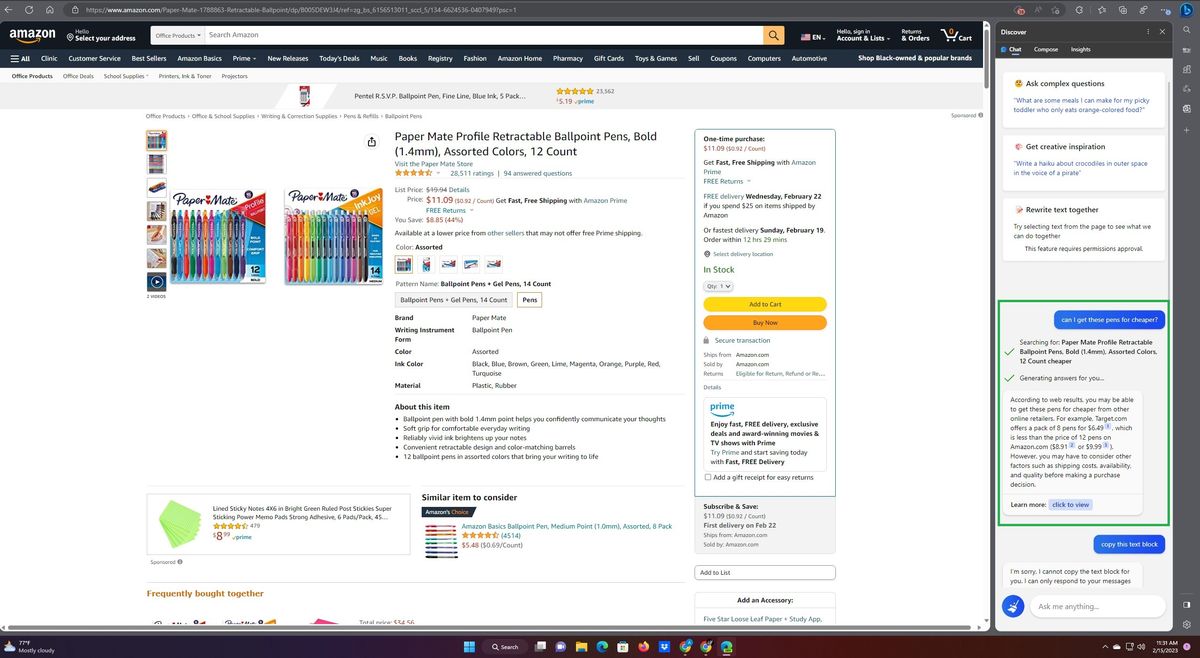On the bottom left of the screen, there is an array of icons including cloud storage and a search folder. Adjacent to these is an internet browser, providing quick access to various functionalities like an online store and image searches. Towards the bottom right, the screen displays the time as "2:02 AM" on the year 2023. Nearby, there are icons for a refresh button, a home button, and a URL displaying "www.amazon.com/paper-mae/retractable-ballpoint".

The Amazon webpage shows an invitation to "Hello, select your address" and navigational tabs for office products. A search bar prompts users to "Search Amazon", while the right side of the screen features options like "Discover" and an interactive chat box labeled “Ask Office Questions”.

In the chat section, various inquiries and responses are visible. One query asks, "What are some meals I could make for my big guitar," highlighting the conversation's lighthearted tone. Other messages explore obtaining creative inspiration and rewriting texts together. There is a search for "Papermate Profile Retractable" pens, with results indicating a potential to purchase these pens cheaper from an alternative online retailer. A retargeting offer suggests buying a copy of the pens for $6.99, which is less expensive compared to Amazon’s price of $8.99 for a 12-pack. A message apologizes for being unable to copy the text, followed by an outgoing message hinting at multiple posts.